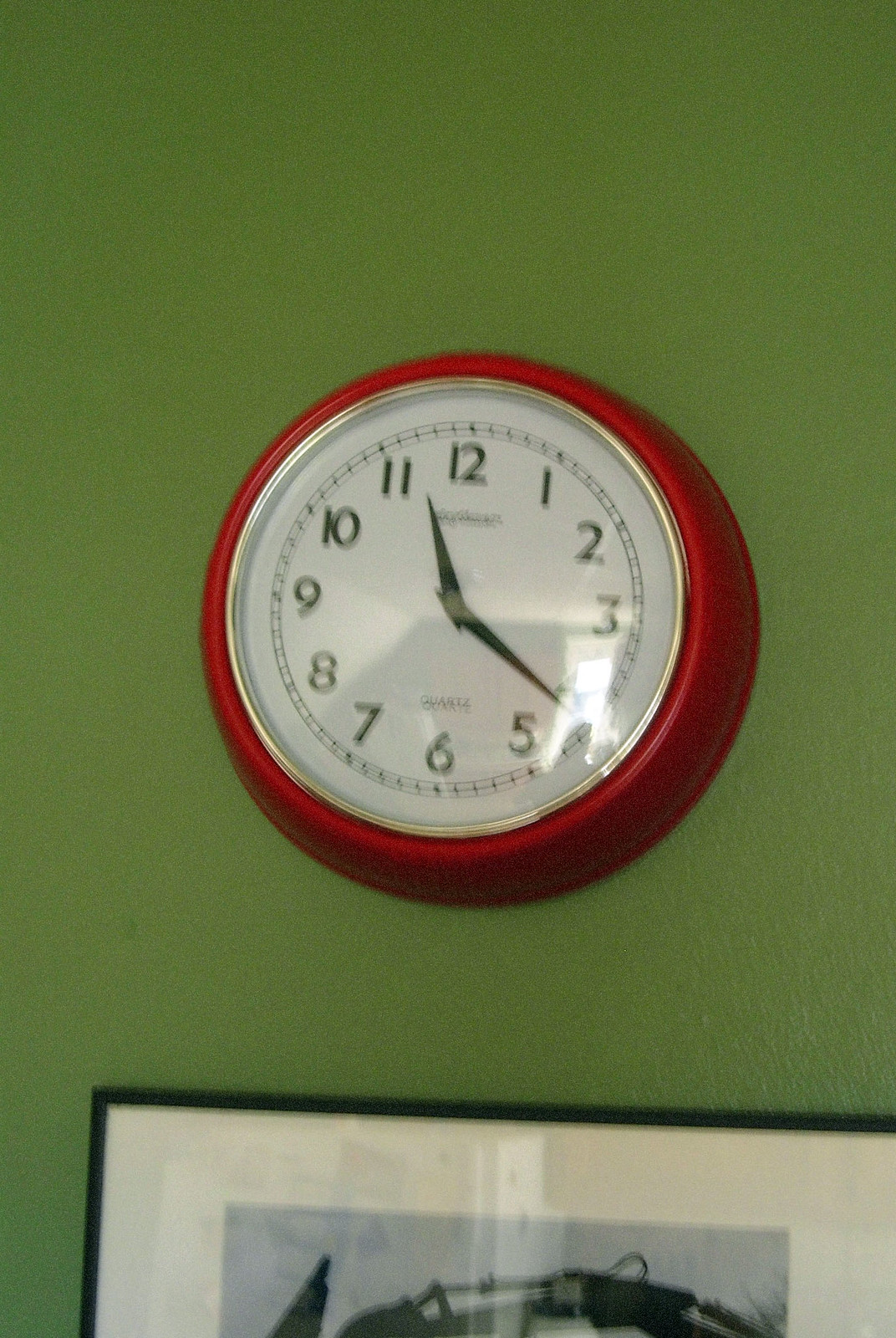This is a blurry, low-resolution image depicting a wall clock prominently centered on a green-colored wall. The clock has a black frame with a red border, and its circular face is white. Black numerals and hands mark the time, with the word "quartz" inscribed in black at the bottom of the clock face. Below the clock, part of a picture frame is visible, though the rest of the frame is obscured in this poor-quality image.